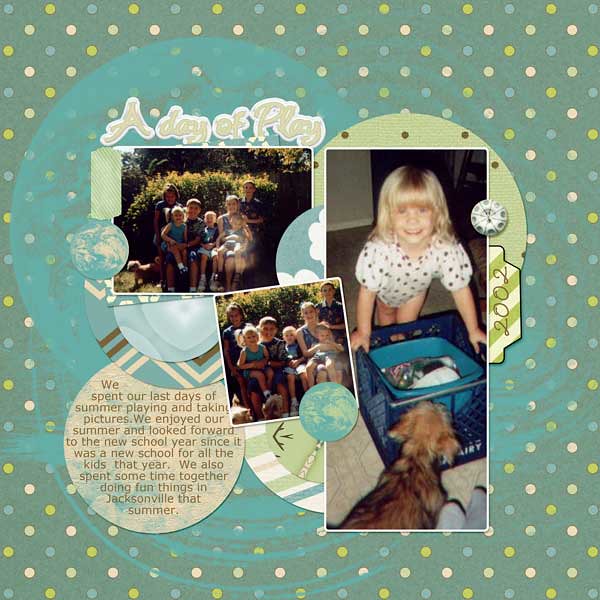The image is a digital scan of a family’s greeting card from 2002, designed with a scrapbook-style layout. The background is dark green, decorated with light blue, gold, and white polka dots that give it the appearance of wrapping paper. The card features three photographs of varying sizes, organized in a square format that is slightly longer than it is wide.

The top left photo, framed by a green circle with "A Day of Play" stylized in white, depicts an outdoor family gathering with four adults and three children of various ages sitting and standing in front of a bush. 

The central photograph, slightly tilted to the left, is a close-up of the same family in the first image. In this photo, a tall man, possibly the dad, stands behind a woman, likely the mom, who is holding an infant and a toddler. To their left, an older man, who could be the grandpa, sits with another toddler on his lap, accompanied by a woman who might be the grandma standing behind them.

The right-hand portion of the card presents a vertical photo of a young blonde girl with shoulder-length hair and bangs. She is indoors, leaning over a blue milk crate with items inside and smiling at the camera. The family’s small brown dog is sniffing at the food on a tray in front of her. Next to this photo, there is a tab labeled "2002."

At the bottom left, within a light tan circle, there is an inscription in a clear printed font: "We spent our last days of summer playing and taking pictures. We enjoyed our summer and looked forward to the new school year since it was a new school for all the kids that year. We also spent some time together doing fun things in Jacksonville that summer."

The card includes additional decorative elements such as images of the globe and an astrological sign circle arrayed like a clock, adding a personalized and nostalgic touch to the family's seasonal memory.